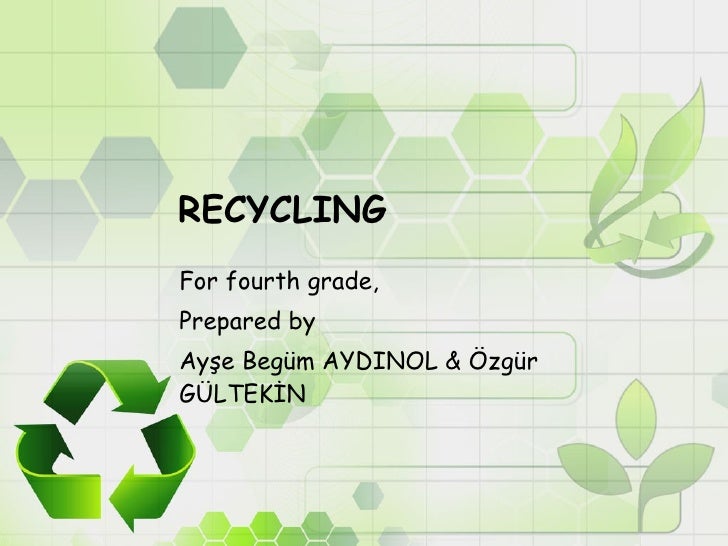The poster is predominantly white with hints of light green, particularly in the upper left corner. A striking feature is the hexagonal honeycomb pattern scattered across the top portion, with hexagons in varying shades of green. The title "RECYCLING" is displayed at the top in bold, black Comic Sans font. Below this, in a softer, non-bold Comic Sans, it states "For 4th Grade" followed by "Prepared By" in a similar style. The credits feature two lines of foreign text that appear to be names, "Ice, Bejum, Idenol" (with "Idenol" in all capital letters) and "Ampersand, Osger, Goldtiken" (with "Goldtiken" in all capital letters). 

In the bottom left corner, there is a green recycling logo composed of three arrows forming a triangle, symbolizing the recycling process. Near the middle right, two green leaves end as arrows pointing towards each other, adding a touch of nature to the design. Additionally, three leaves are featured at the bottom of the poster. The overall background fluctuates between white and light green, enhancing its environmental theme.